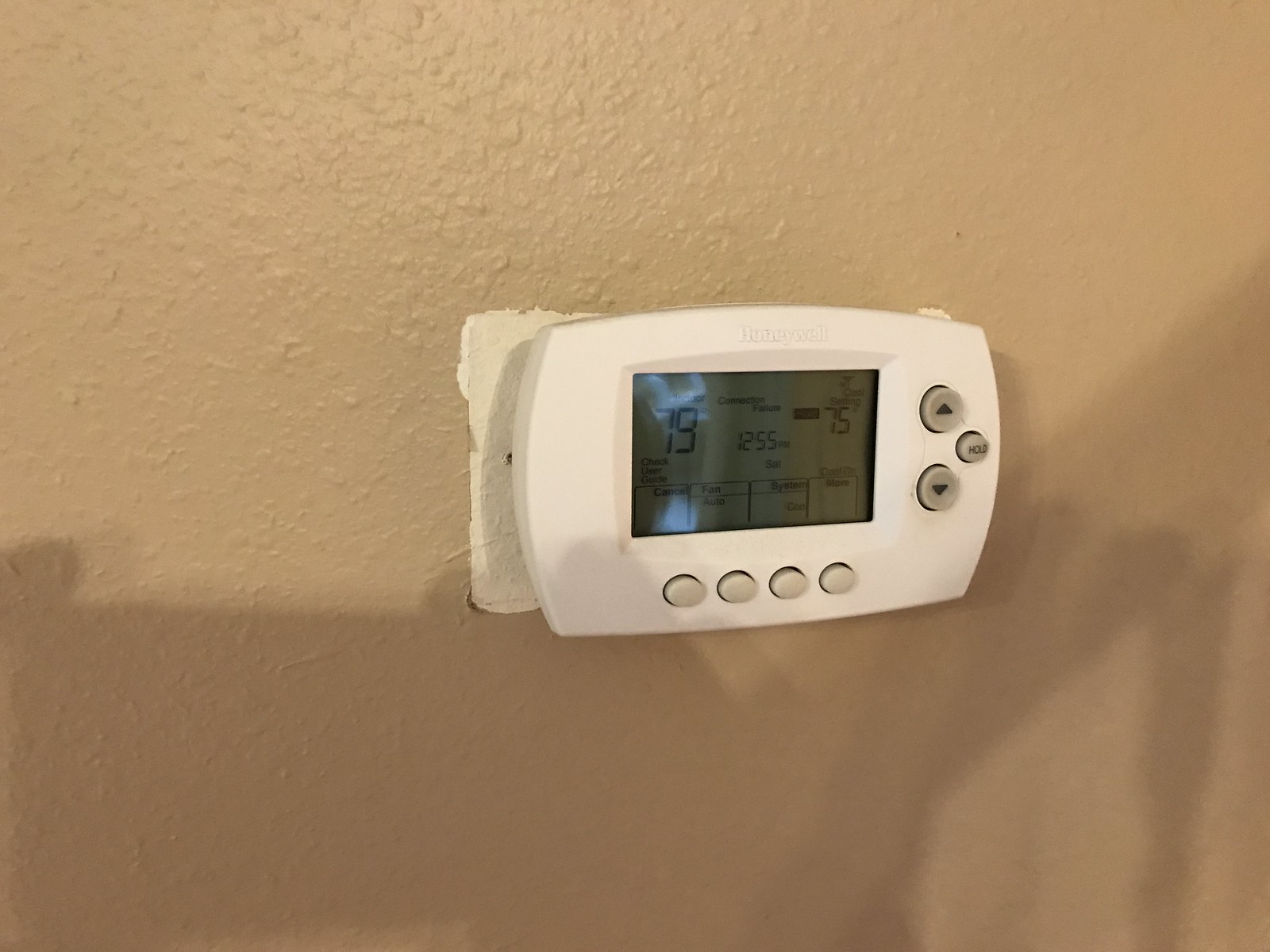In this detailed photograph of a household thermostat mounted on a beige-painted wall, the contrast between the new and old devices is evident. The wall reveals a cream-colored patch, indicating where the previous, larger thermostat had been placed prior to the current installation. The newly installed thermostat, a sleek white plastic model by Honeywell, features a digital screen that displays the current indoor temperature, time, and date. Positioned below the screen are four labeled buttons. From left to right, the labels above these buttons read: "Cancel," "Fan" (currently set to auto), "System" (showing cool), and an unreadable label, likely "Menu." To the right of the digital screen, three additional buttons are aligned vertically: an "Up" button, a "Down" button, and between them, slightly off-center, a "Hold" button. This programmable thermostat exemplifies modern climate control technology amidst a traditional home setting.